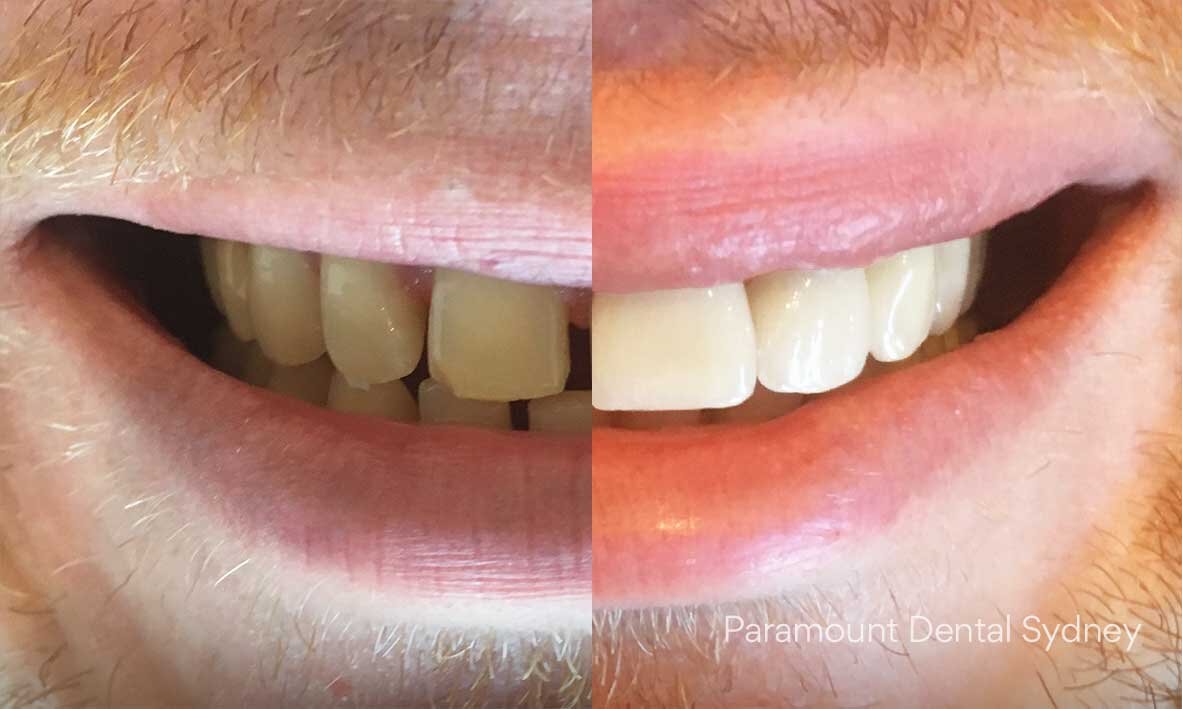This image, attributed to Paramount Dental Sydney, showcases a compelling before-and-after comparison of dental work. The split-screen photo features a close-up of a man's smile, divided into two halves. On the left side, representing the "before" shot, the lighting is dim, highlighting the man's discolored, gapped, and slightly crooked teeth. His facial hair, including slight stubble, is consistent across both sides, indicating it's the same individual. On the right side, the "after" image is brightly lit, emphasizing the dramatic transformation: the teeth are now perfectly aligned, brilliantly white, and free of gaps or imperfections, suggesting the application of caps or crowns. The stark contrast between the two halves underscores the effective dental procedures performed at Paramount Dental Sydney, as indicated by the white lettering in the right lower corner of the image.